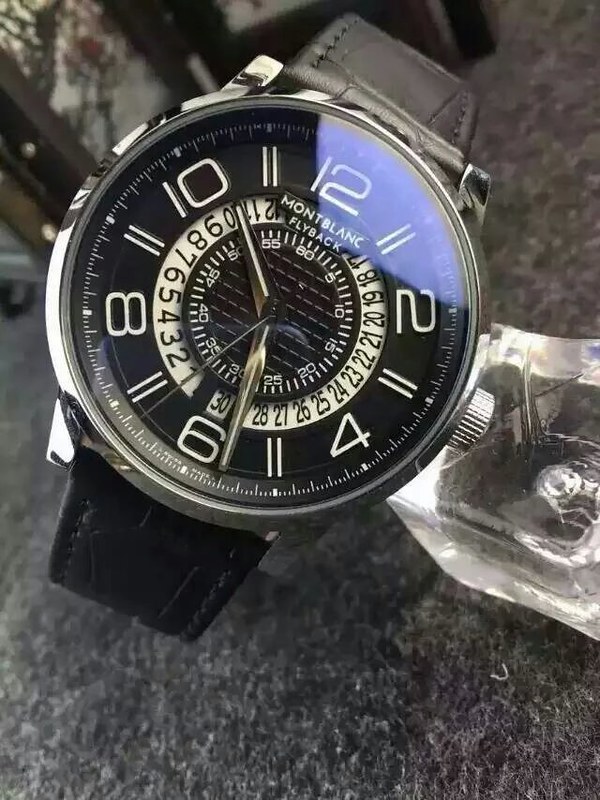This detailed photograph captures a sophisticated Mont Blanc Flyback wristwatch. The watch face features a prominent black background with even numbers (12, 2, 4, 6, 8, 10) in white, while the odd numbers are denoted by two narrow vertical dashes resembling the Roman numeral II. The watch is equipped with silver, arrow-like hour and minute hands, which include a white stripe. The hour hand points to 10, the minute hand is between 5 and 6, and the seconds hand is positioned between 7 and 6. Just below the 12 o’clock mark, the text "Mont Blanc Flyback" is clearly visible in white. The dial comprises multiple layers, with the outermost being black with white numerals, followed by an inner white ring of smaller numbers from 1 to 30, and a central circle showing numbers from 1 to 60. The watch's strap appears to be black leather or faux leather. The watch rests against a clear, cube-shaped stand that resembles a block of ice. The background is a black-and-gray carpet with a fuzzy texture, and parts of what might be a flowered pattern and a door or cabinet are faintly discernible.